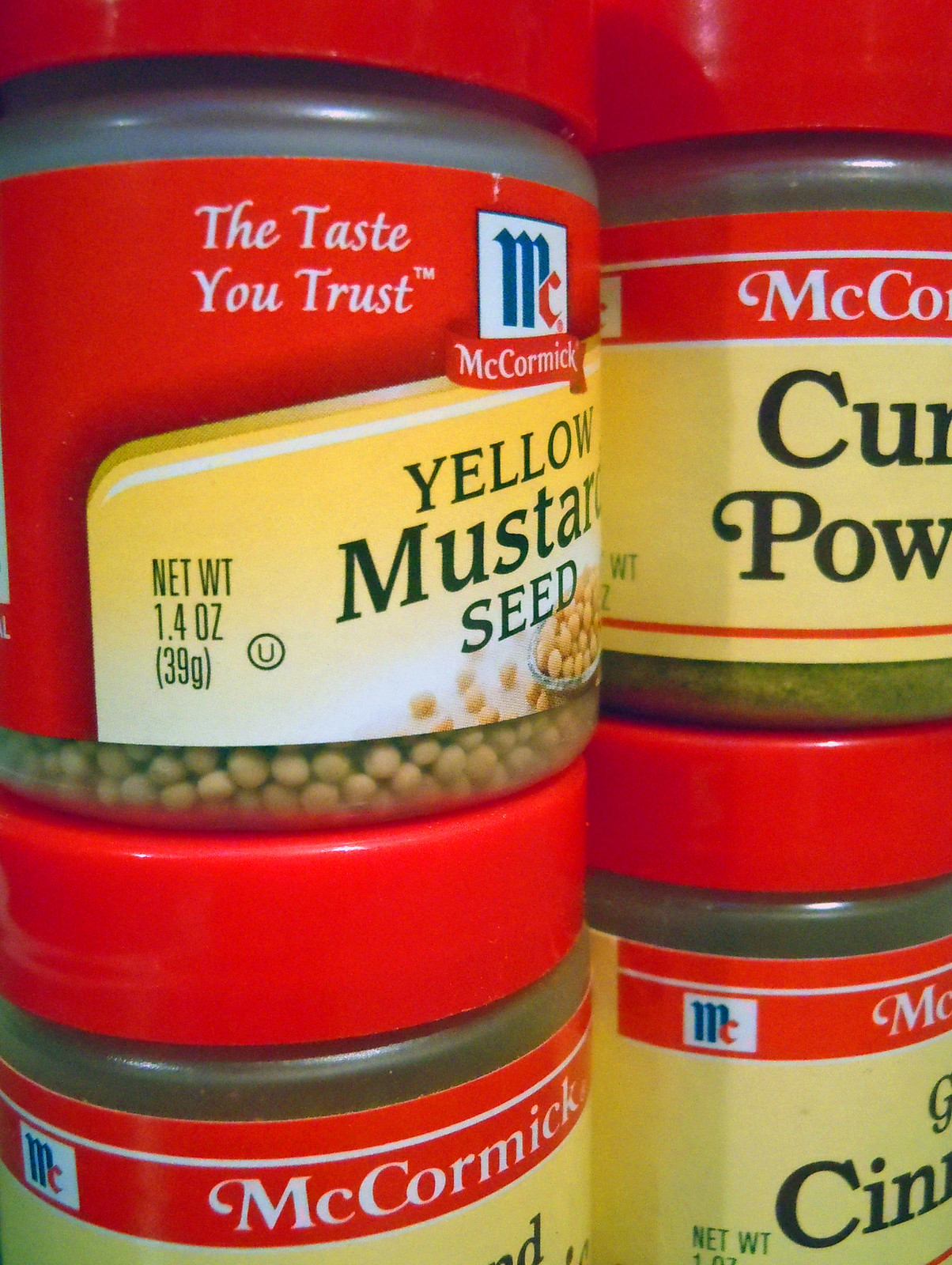The image depicts a collection of various spice jars, each bearing distinctive labels and associated colors. On the top of the central jar, the phrase "The Taste You Trust" is prominently displayed. Below this, there's a white square featuring a letter 'C' in blue and red hues situated in the corner. The label beneath states "Yellow Mustard Seed," detailing its contents.

To the right of the mustard seed jar, there is another jar labeled "Cumin Powder." The side of this jar reveals a view of the spice itself, showing a brown powder. Below this jar, the label specifies "Ground Cinnamon."

On the left side of the display, another jar is partially visible, characterized by a red label typical of the McCormick brand. The exact spice in this jar isn't clear from the description, but it follows the recognizable design with a small blue and red square logo. The "Yellow Mustard Seed" jar is further described as having tiny yellow seeds visible within. 

Overall, the scene captures an organized collection of McCormick spice jars, highlighting their branded labels and the spices contained within them.